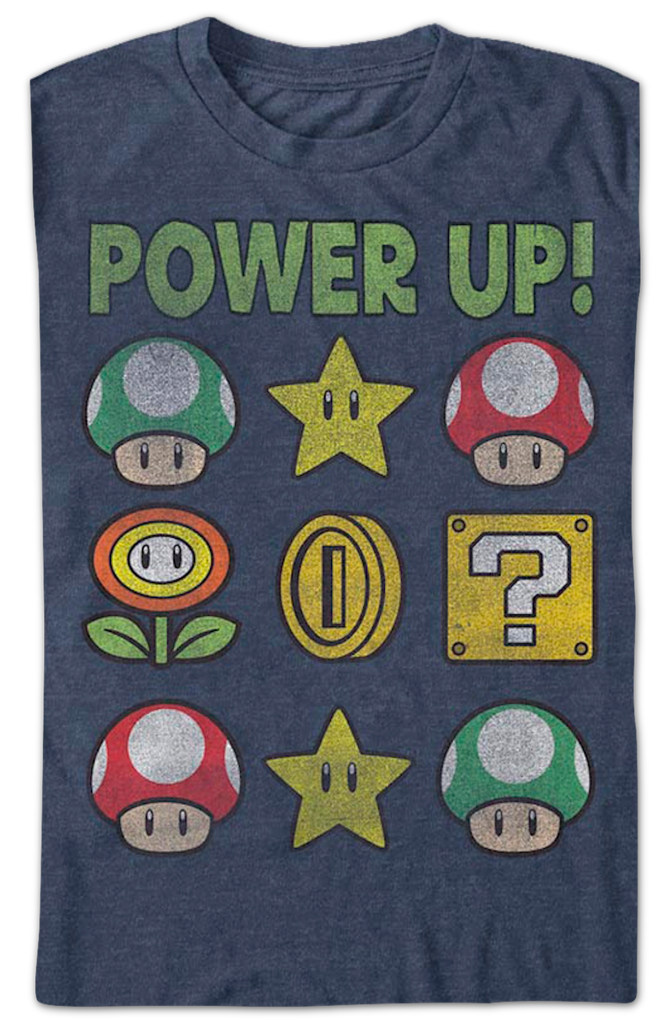The photograph captures a folded, light to mid-tone grayish blue t-shirt, appearing pre-washed for a vintage texture. The shirt's design features the phrase "POWER UP!" in a bold, yellow-green, retro-styled font across the chest. Below the text, nine iconic symbols from the Mario franchise are arranged in a 3x3 grid, giving the design a nostalgic feel with a slightly rubbed-off print for an aged effect. The top row includes a green 1-UP mushroom on the left, a yellow star in the center, and a red mushroom to the right. The middle row features a fire flower on the left, a coin in the center, and a yellow question mark block on the right. The bottom row repeats with another red mushroom on the left, another star in the center, and a second green 1-UP mushroom on the right. Though folded, the t-shirt’s round neckline and partial front design are clearly visible, suggesting a casual, stylish piece that showcases beloved elements of the Mario universe.